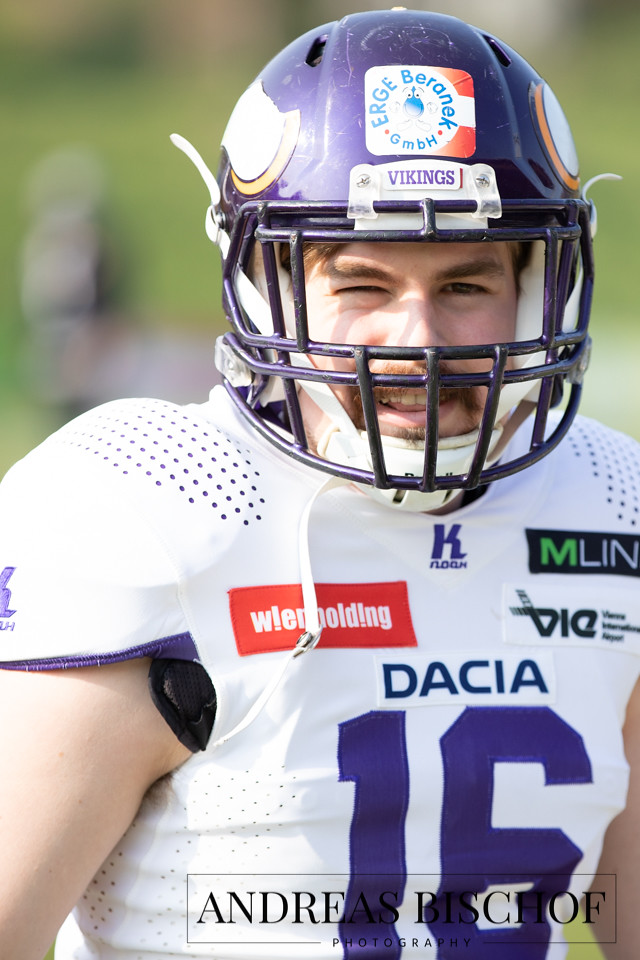The photograph is a full-color, horizontally rectangular image taken outdoors on a bright sunny day at a sports event. The focus is a Caucasian adult male football player who plays for the Minnesota Vikings, wearing the number 16 on his white away uniform. He has a purple helmet with the word "Vikings" near the faceguard and various stickers and sponsor logos, including a distinctive red, rectangular one in white font, and a letter 'K' with unknown text beneath it. The image captures him from just below his chest upwards, with one arm partially visible and the other obscured. The player, squinting with one eye half-closed, appears to be attempting a smile, revealing his teeth. The sunlight reflects off his helmet and illuminates the scene from the left side. At the very bottom of the photograph, there is bold, black text reading "Andrew Bischoff photography,” identifying the photographer.